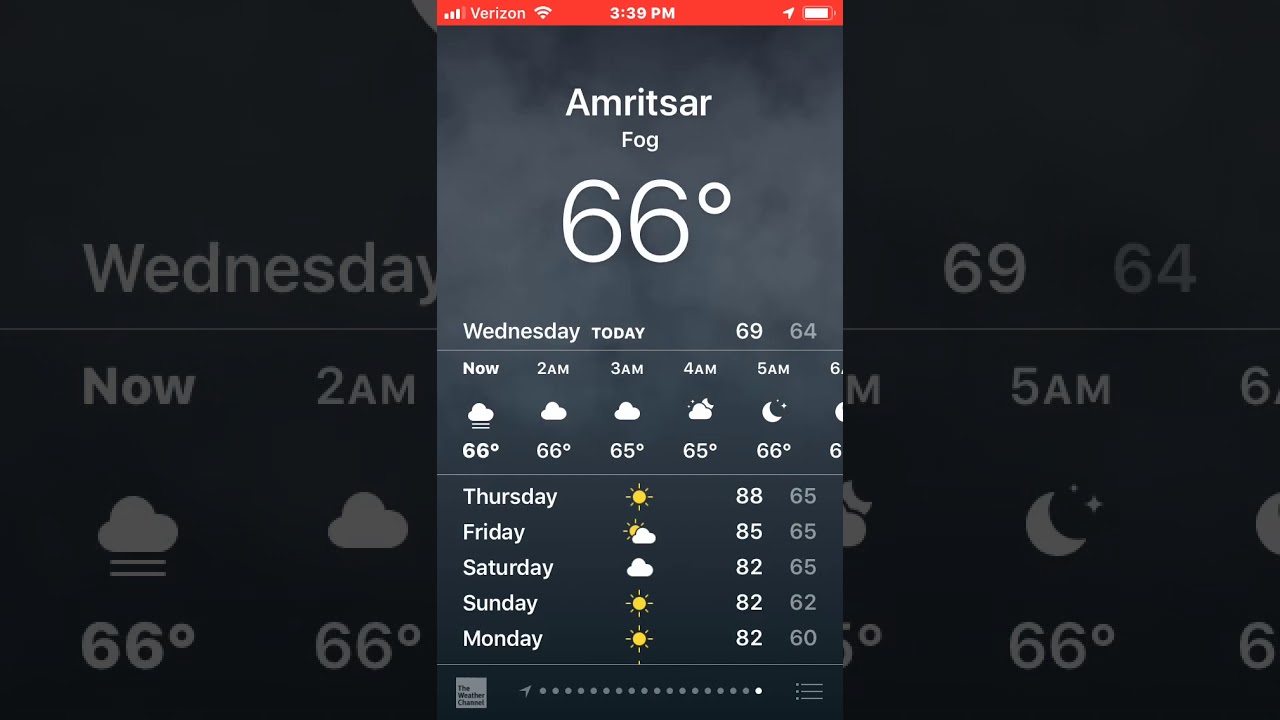The image portrays a smartphone screen displaying a weather report. 

In the center of the screen, a section provides detailed weather information for Amritsar: "66°F, Fog." At the top of this section, a red line displays the Verizon logo, signal strength, and the time, which is 3:39 p.m. Additional icons for Wi-Fi and battery status are also visible.

Below the primary weather report, the forecast for the week is listed, including temperatures and weather conditions for Wednesday (69/64°F), Thursday, Friday, Saturday, and Sunday. The background also features a darker overlay depicting a broader forecast view.

At the bottom of the screen, a "The Weather Channel" logo is accompanied by navigational dots, indicating that there are multiple pages available, with the display currently on the last (15th) dot. 

The entire scene is set against a black backdrop, creating a slightly mysterious or 'shady' ambiance.